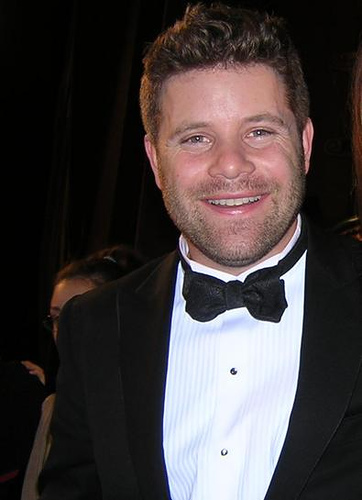This photograph features Sean Astin, positioned slightly to the right of center. He is smiling and dressed in a classic black tuxedo with a black bow tie and a white shirt adorned with silverish black buttons. Sean's medium-length brown hair is wavy on top and shorter on the sides, brushed off his forehead. He sports a light beard and mustache, giving him a distinguished appearance. The image captures him from the top of his head to just below the chest, with a slight glimpse of his left shoulder visible. 

In the background, over Sean's shoulder, a woman with dark hair pulled back into a ponytail can be seen. She has dark eyebrows and is wearing a gray shirt, with just part of her head and one eye visible. Additionally, another person's hand rests on her right shoulder, adding a subtle layer of interaction within the scene. The backdrop consists of curtains on both the left and right sides, suggesting an indoor, possibly formal, setting.